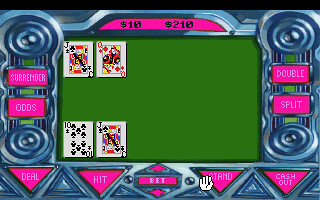This screenshot captures an intense moment in a virtual game of Blackjack. At the center, a green playing table sets the stage, surrounded by various controls arranged in a U-shape configuration. These controls, presented in dark pink with white text, are accented by blue geometric decorations, including triangles and circles. At the top of the screen, the player's currency is displayed, showing amounts of $10 and $210.

In the gameplay area, the top cards revealed are the Jack of Clubs and the Queen of Diamonds, while the bottom cards are the Ten of Clubs and another Jack of Clubs. The available controls include options to Surrender, place Odds, Deal, Hit, Bet, Stand, Cash Out, Split, and Double. A hand cursor is prominently hovering over the 'Stand' button, indicating the player's next potential move in this strategic game.